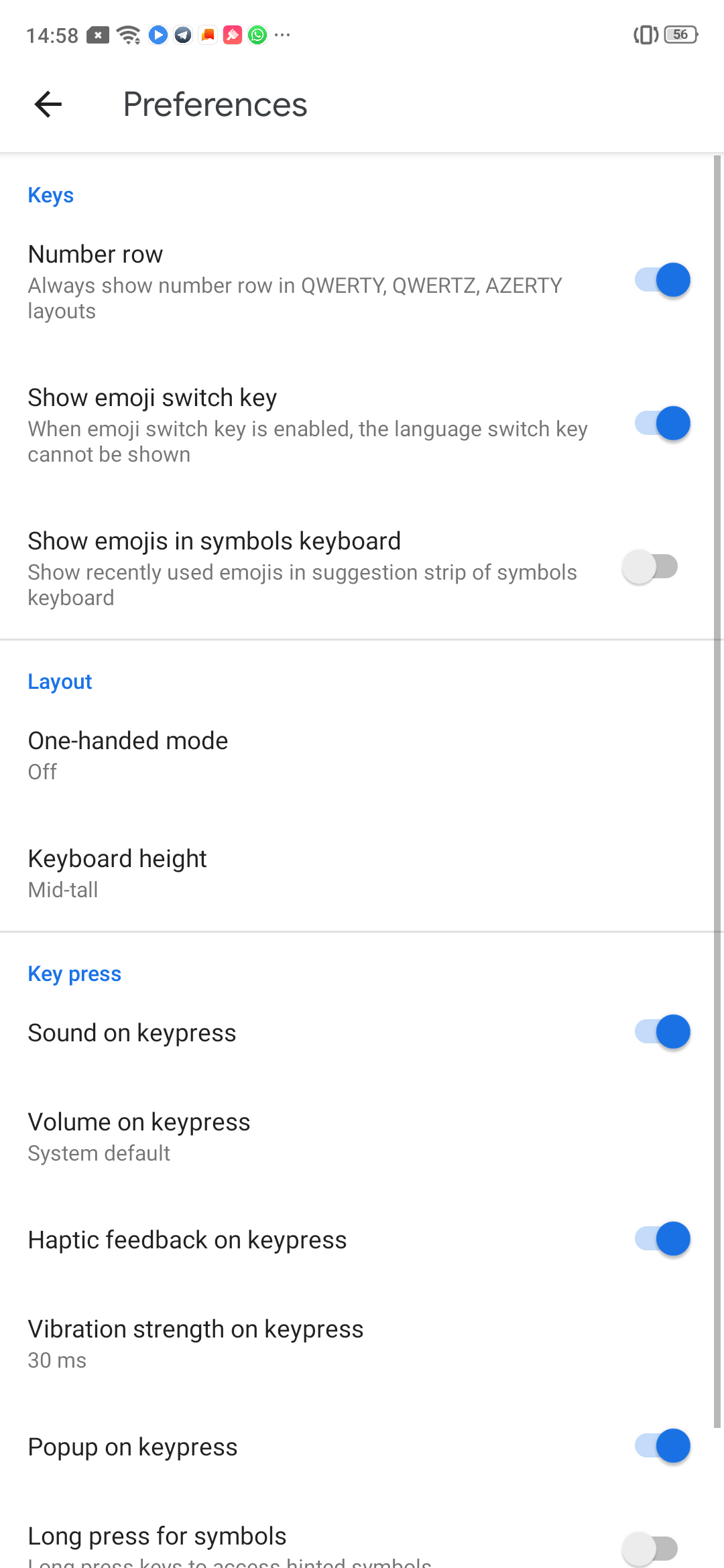**Detailed Caption:**

The image is a screenshot taken from a phone, characterized by a white background with black text and various icons. 

**Top Section:**
- In the top left corner, the time is displayed as "14:58".
- To the right, a black box features a white icon resembling an "X".
- Adjacent to this is the Wi-Fi strength bar.
- Next in line is a blue circle with a white arrow pointing to the right.
- Following this is a black circle containing an indiscernible white icon.
- A red icon, which is difficult to make out, appears next.
- Accompanying these is a red box with a white dot inside.
- A green circle with a white circle in its center follows.
- Three small horizontal dots trail next to it.
- The right-hand side hosts a phone icon, outlined in black to indicate vibrations.
- Next to it, a battery icon, white with a black outline, displays "56".

**Main Content:**
- Below these indicators, a black left-pointing arrow precedes the word "Preferences".
- A small gray line separates this from further content.

**Preferences Section:**
1. **Keys Section (in Blue):**
   - "Number row"
   - Text stating: "Always show number row in QWERTY, QWERTZ, AZERTY"
   - "Layouts" followed by a blue bar with a blue circle on the right.
2. **Emoji Switch Key Section:**
   - "Show emoji switch key"
   - Explanation: "When the emoji switch key is enabled, the language switch key" (incomplete due to cutoff).
   - Another blue bar with a blue circle to the right.

3. **Emoji Preferences:**
   - "Show emojis in symbol keyboard"
   - "Show recently used emojis in suggestion strip of symbols"
   - The word "Keyboard" followed by a gray bar with a gray circle on the left.

4. **Layout Section (in Blue):**
   - "One-handed mode" indicated as "Off"
   - "Keyboard height" specified as "Mid-tall"

5. **Key Press Section (in Blue):**
   - "Sound on key press" matched by a blue bar with a darker blue circle on the right.
   - "Volume on key press" specified as "System default".
   - "Haptic feedback on key press" also accompanied by a blue bar with a darker blue circle on the right.
   - "Vibration strength on key press" denoted as "30 ms".
   - "Pop-up on key press" with a blue bar and a darker blue circle on the right.
   - "Long press for symbols" but the text is partially cut off at the bottom.

The detailed description captures the content and structure of the phone screenshot, providing a comprehensive overview of the UI elements and settings visible.